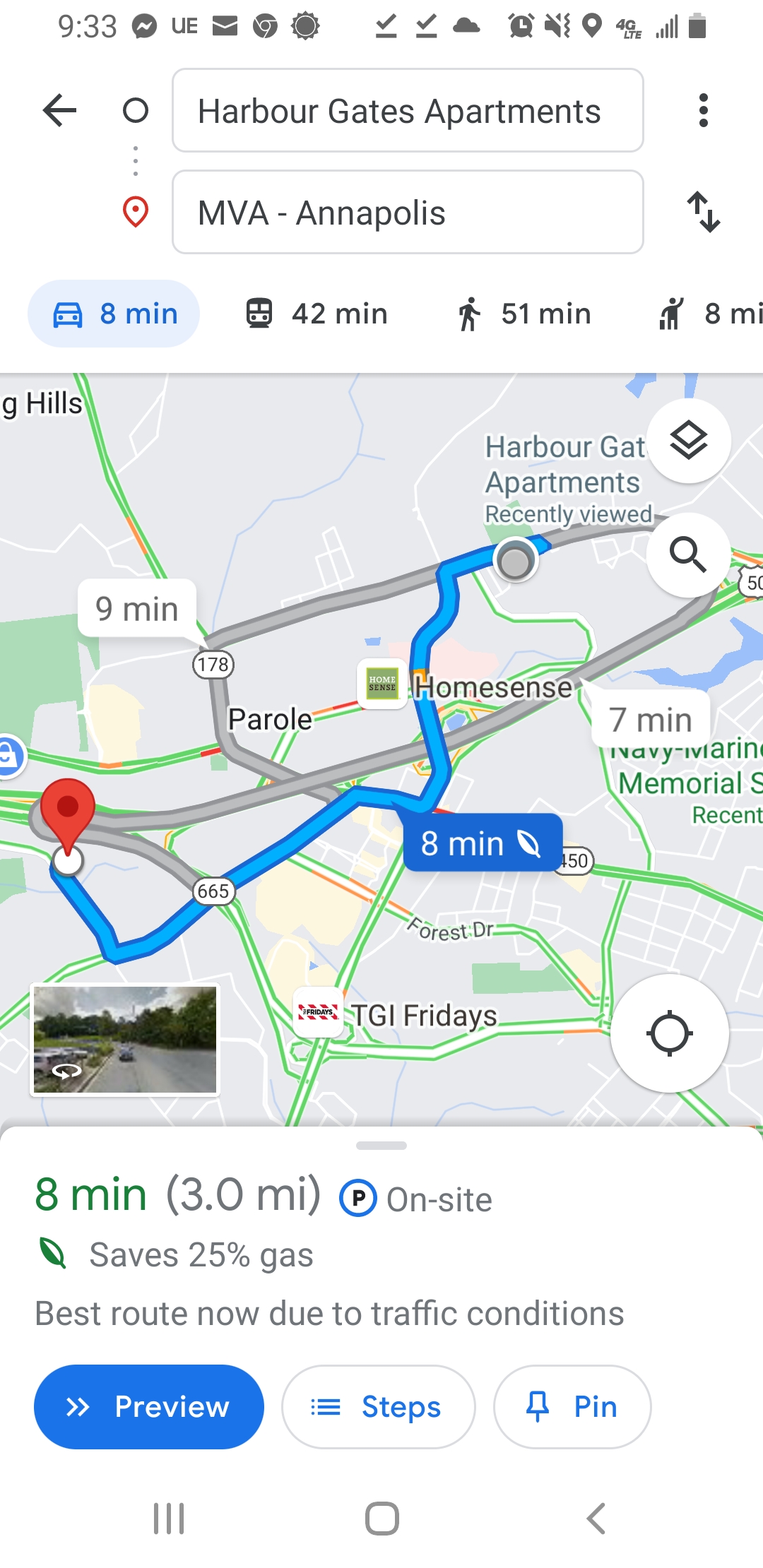This is a detailed screenshot of Google Maps from a smartphone, showing directions from Harbor Gates Apartments to MVA-Annapolis. The daytime interface features a white and black UI, along with various typical interface icons at the top of the screen, including clock, notification logos, mail, Chrome, weather, alarm, signal bars, and battery life. The navigation data at the top indicates that the trip by car takes 8 minutes to cover 3 miles, while public transport takes 42 minutes, and walking takes 51 minutes.

The route is visually represented in blue on the map, indicating an optimal path with no delays, while a street view image of the destination is visible in the bottom left corner. Additional on-screen details include "best route now due to traffic conditions," an option to view the driving steps, and a note that this route saves 25% on gas. A blue button at the bottom of the screen allows users to preview the route.